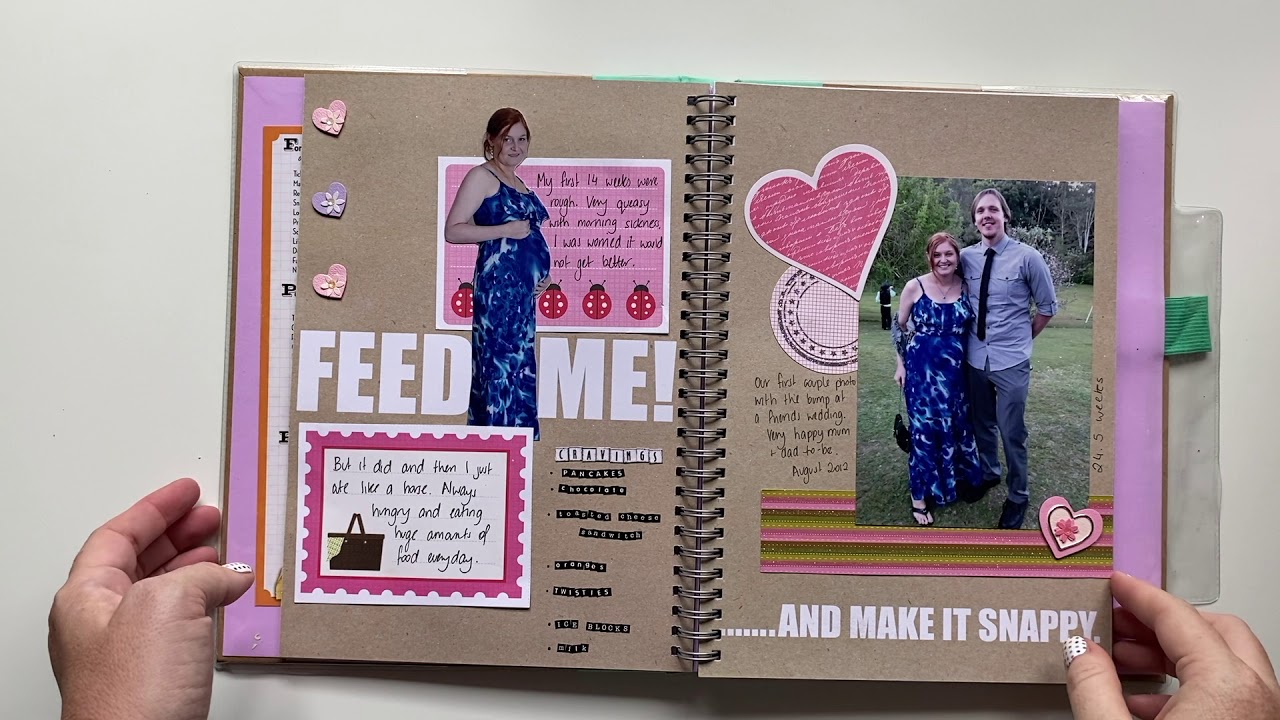This image depicts an open spiral-bound journal, possibly a baby scrapbook. The journal has brown pages accented with pink elements and is being held open by a person, showing two detailed and whimsical entries. On the left page, bold letters declare "FEED ME," above a photograph of a young, pregnant woman with red hair, adorned in a blue tie-dye sundress, holding her belly and looking at the camera. The caption below details her experience during the first 14 weeks of pregnancy, mentioning difficulties with morning sickness and subsequent cravings for foods like pancakes, oranges, twisties, ice blocks, chocolate, loaded cheese sandwiches, and milk. The page is decorated with foam hearts, flowers, and ladybug stickers.

On the right page, the phrase "AND MAKE IT SNAPPY" is prominent. The accompanying photo shows the same woman and a man, presumably her husband, wearing a grey long-sleeve shirt, black tie, and jeans, standing together at a friend's wedding, smiling and joyful. This first couple's photo with her baby bump is historicalized as August 2012. The page is further adorned with a pink heart sticker in the top left corner, adding to the scrapbook's loving and celebratory theme.